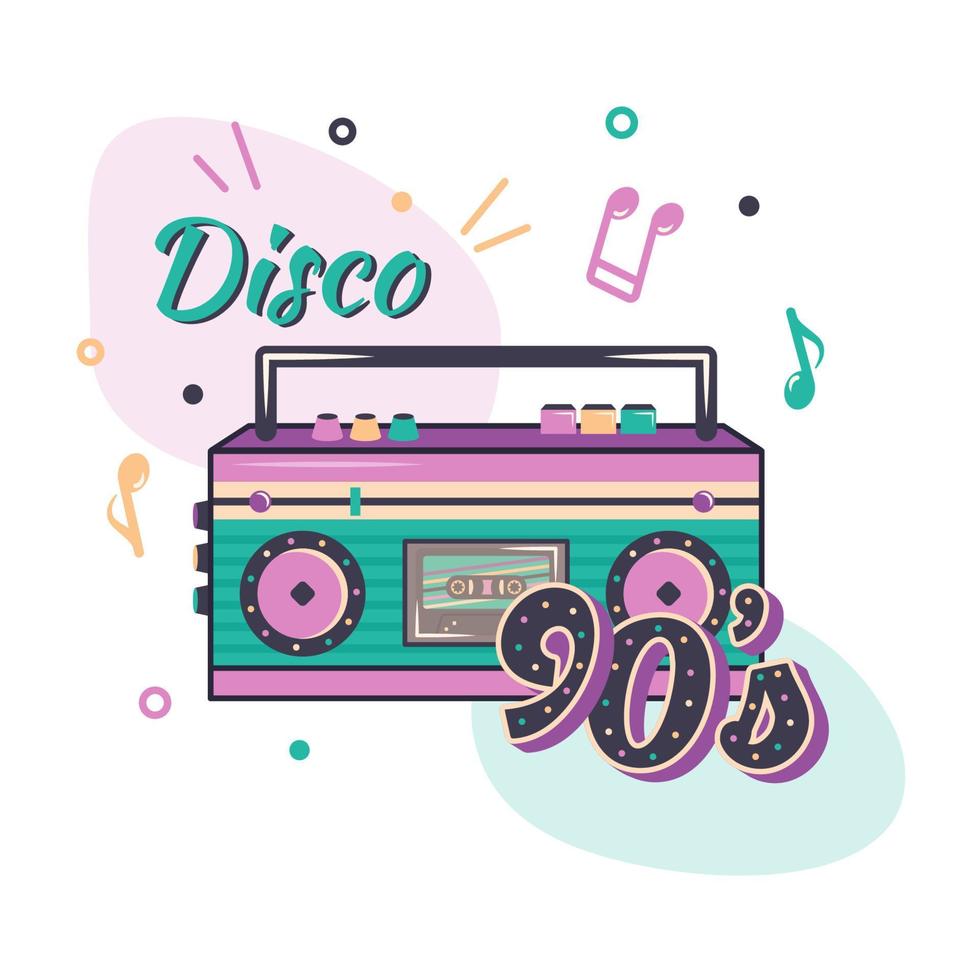This cartoonish illustration features a multi-colored, pastel boombox prominently in the center, adorned with shades of purple, pink, and green stripes, complete with a tape in the deck and a raised handle. The boombox's front showcases two large purple speaker circles and an array of colorful buttons at the top—three on the left (round and in purple, peach, and green) and three on the right (square and in matching hues). Set against this vibrant backdrop, the word "disco" bursts out in a big pinky-purple blob in the top left-hand corner, while "90s" is inscribed within a blue blob in the bottom right-hand corner. Surrounding the boombox, multi-colored musical notes in green, purple, and peach, as well as various circles and dots, add a dynamic sense of rhythm and movement. The overall aesthetic, reminiscent of 90s stickers ideal for decorating Chopper Keepers, encapsulates a playful nostalgia with its soft pastel hues and lively patterns, celebrating an era of portable music and carefree fun.